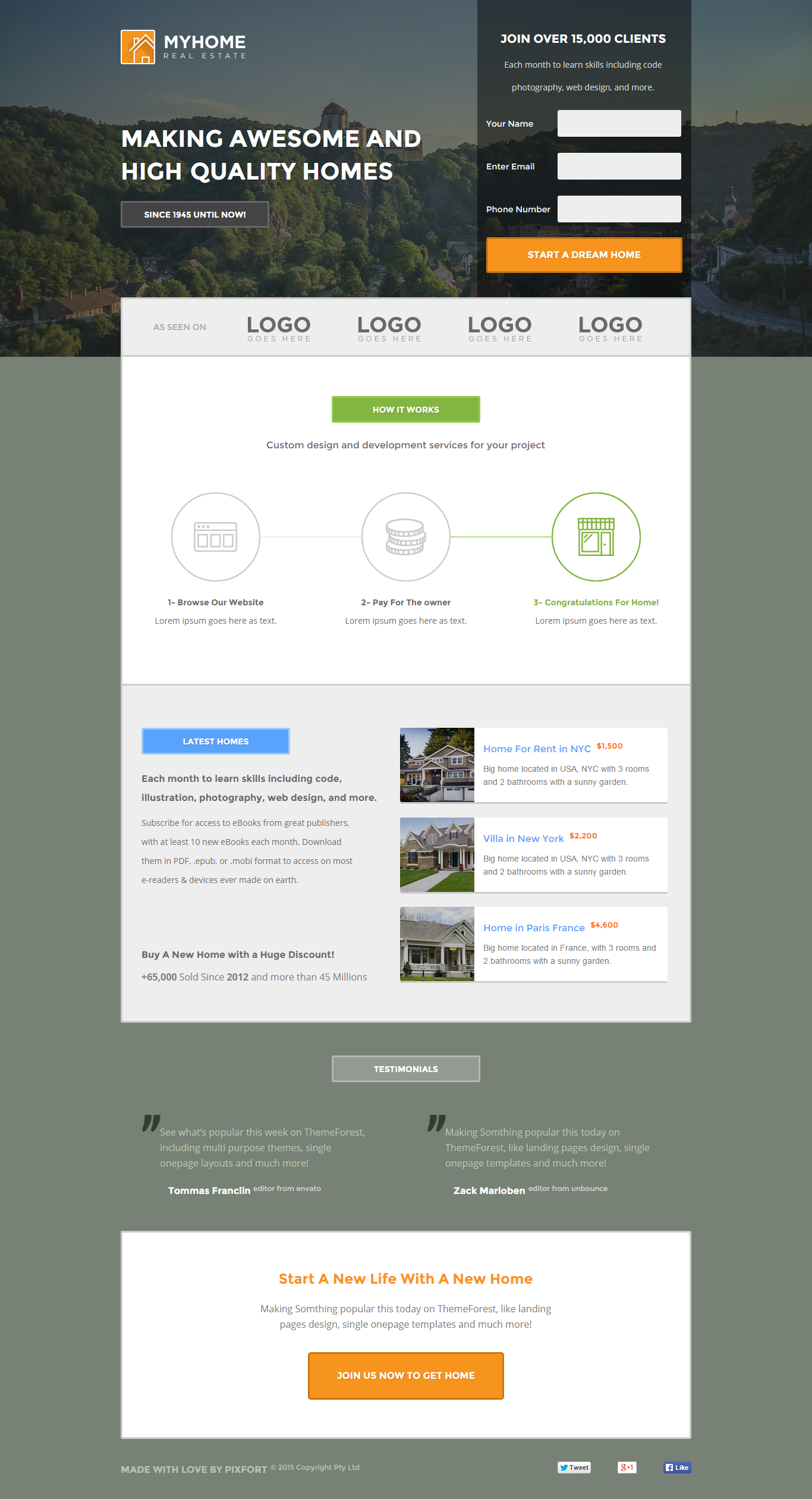In the image, the header reads "MY HOME" at the top, where an orange block with an icon of a home appears next to the text. Beneath this, "MAKING AWESOME AND HIGH-QUALITY HOMES" is prominently displayed in white capital letters. The background of the image features a filtered, gray-toned photograph that shows a picturesque view of green Appalachian mountains, adding a serene touch. The middle section invites viewers to "JOIN OVER 15,000 CLIENTS," accompanied by three editable white text boxes and an orange call-to-action button. Further down, the acronym "L-O-G-O" is repeated in four distinct locations, followed by a green button. Towards the bottom section, there are three circles under which lies an icon, followed by three images of homes, each accompanied by a brief description on the right. The image concludes with a gray button at the very bottom.